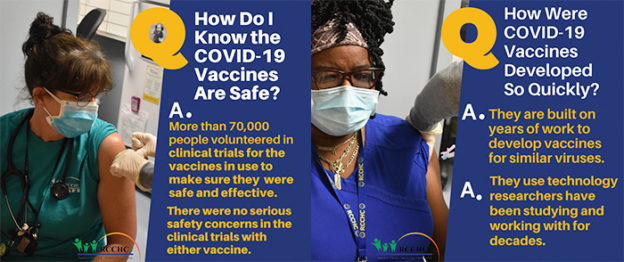The image features a purple background with two primary sections. On the left side, there's a photograph of an African American woman wearing a protective mask while receiving a vaccination. Adjacent to this image, a prominent purple box is visible with a large yellow "Q" in the corner, presenting text that addresses common questions about COVID-19 vaccines.

The first question reads, "How do I know the COVID-19 vaccines are safe?" The respective answer explains that over 70,000 participants took part in clinical trials for the vaccines currently in use, ensuring their safety and efficacy. No serious safety concerns emerged during these trials.

Additionally, the image includes a second photograph of an African American woman, also masked, receiving her vaccine. This is accompanied by another important question: "How were COVID-19 vaccines developed so quickly?" The answer clarifies that the development of these vaccines is based on years of research concerning similar viruses and leverages decades of established technology. It emphasizes that the vaccines were not hastily created, but are a result of long-term scientific endeavors.